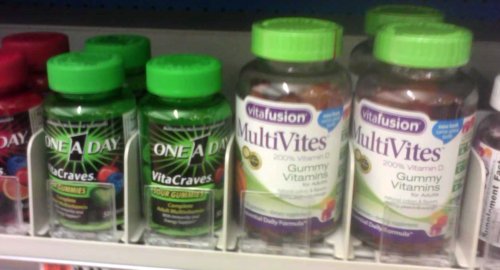The photograph depicts a shelf in a store, showcasing a variety of vitamins and supplements neatly organized behind a white plastic separator to prevent them from falling. The shelf itself is a greyish-white color. On the far left, there's a partially visible bottle with a red cap and label, which displays the word 'DAY' in white text. Adjacent to this is a set of two identical green-capped bottles with black and green labels that read 'One-A-Day VitaCraves.' These labels feature a black number '1' radiating green sun rays and mention 'Sour Gummies.' To the right, the largest product on the shelf is a clear bottle with a light green cap. It has a white label with purple text reading 'VitaFusion MultiVites Gummy Vitamins.'